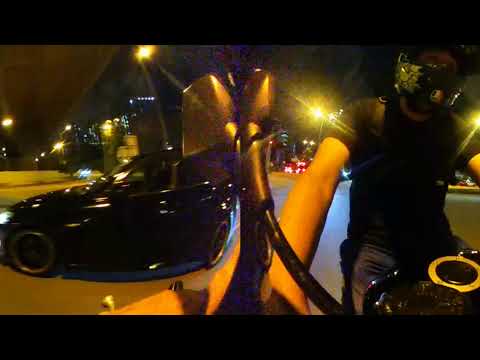In the nighttime city streets illuminated by streetlights, a young motorcyclist wearing a black helmet with a green design, a short-sleeve black t-shirt, and blue denim jeans rides a sleek black motorcycle. His arms are outstretched, and a camera is clipped onto the motorcycle’s windshield, facing toward him, capturing the moment. As he glides on the asphalt, he is closely accompanied by a black sedan, which appears slightly distorted in the image. There's a bright light shining between the motorcyclist and the car, casting an intriguing glow. In the background, distant red taillights and scattered bright lights add depth to the scene, with hints of a gas station on the right, contributing to the urban nighttime ambiance.